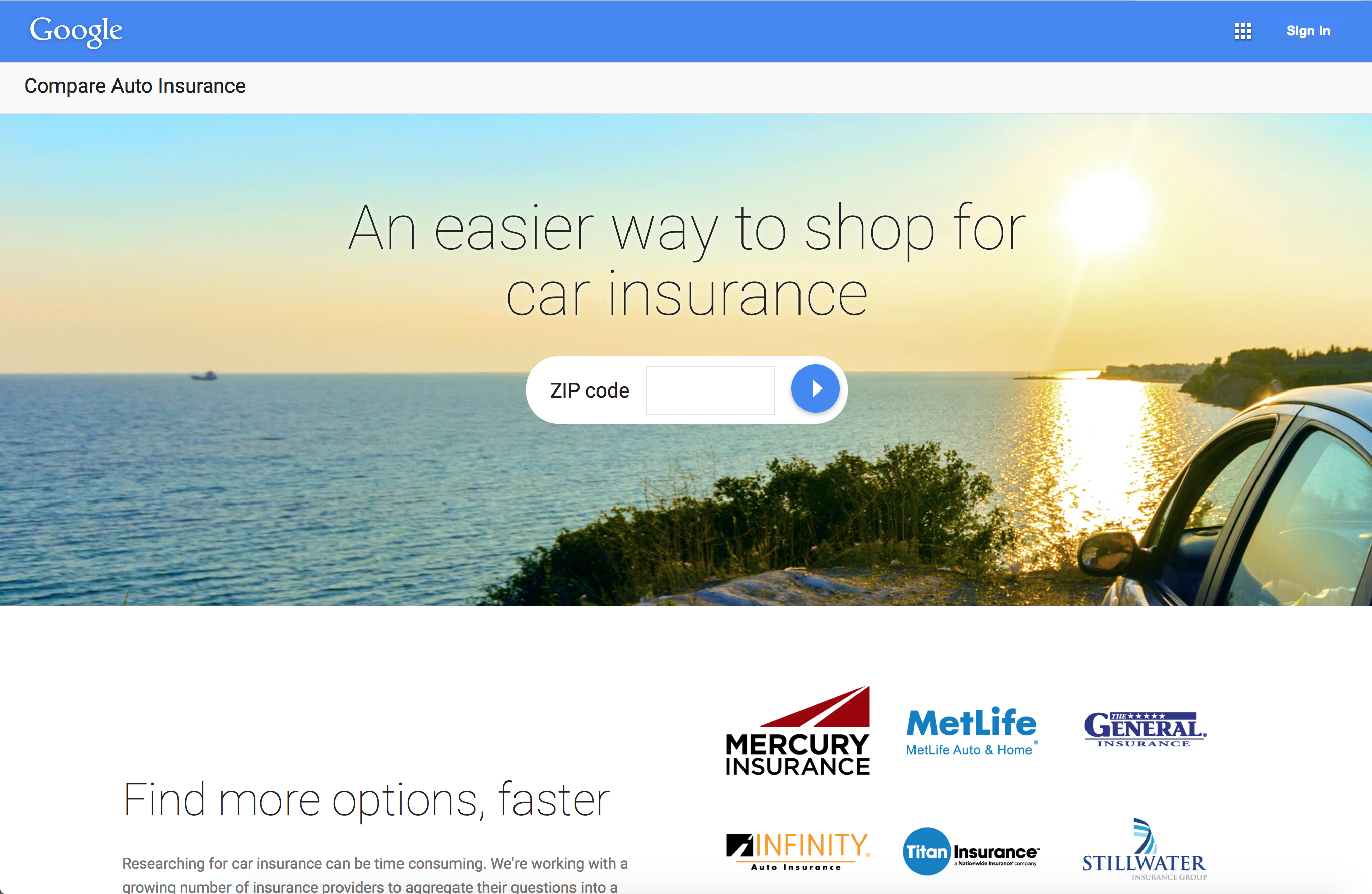Screenshot of Google Auto Insurance Comparison Service

The screenshot features a Google service designed to simplify the comparison of auto insurance options. Against a white background with predominantly black text, this interface provides a streamlined way for users to shop for car insurance.

At the top of the screenshot, the inverted white Google logo is prominently displayed beside a "Sign In" button located on the top left. The layout is divided into two main sections. The upper half showcases a serene image of a car parked by a scenic body of water at sunset, although it is unclear whether the water is a lake or the ocean. The headline reads, "An easier way to shop for car insurance," encouraging users to enter their zip code to initiate a search for insurance rates.

The bottom half of the page is devoted to explaining the functionality of this comparison engine. It describes how the service aims to help users find more insurance options quickly by aggregating various questions into one comprehensive form, subsequently providing a range of rates from different providers. The logos of six participating insurance companies are displayed: Mercury Insurance, MetLife, The General, Infinity, Titan, and Stillwater Insurance.